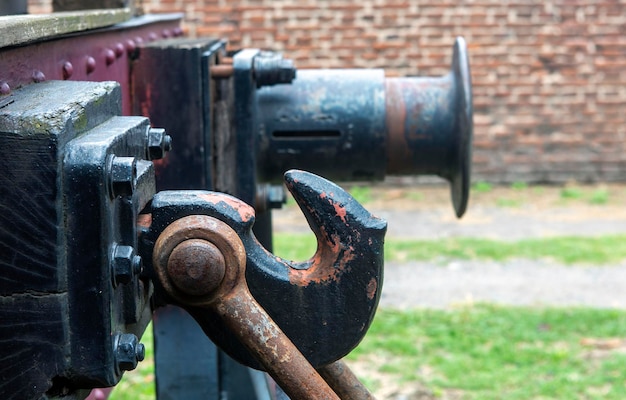The image showcases a detailed close-up of a metal machinery component situated outdoors. The focal point is a visible metal hook-like object mounted within a square peg area surrounded by multiple bolts—three discernible from the front and presumably another three in the back. This square metal piece is layered and connected to a longer section of red steel, distinguished by a line of rounded bolts along its top. The machinery includes various elements made from black, red, and dark gray steel, featuring a prominent rusty lever and a hollow tube. The backdrop reveals a blurry, red brick wall and a patch of asphalt with some weeds, indicating the image was taken outside. A road and a field of grass in the foreground add context to the surroundings.